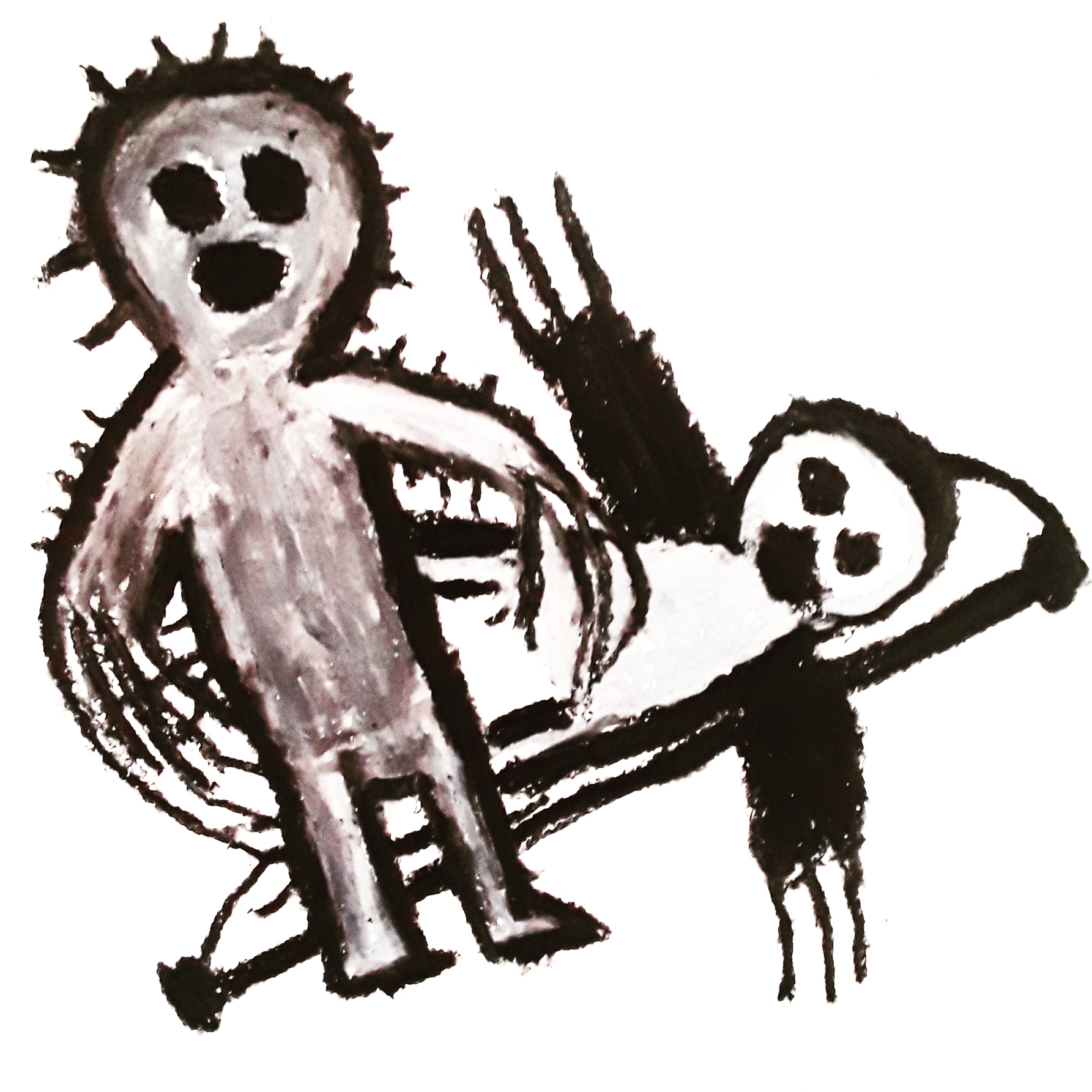The artwork is a crude, rudimentary drawing, possibly made with charcoal or black crayon, featuring two figures with thick, smudged lines and an overall child-like, unrefined style. The figure on the left stands upright, depicted in a gray color with a spiky head and very minimalistic features - two large, black holes for eyes and a large black hole as a mouth. His arms and fingers are exaggeratedly sharp, almost claw-like, outlined heavily in black. Behind this figure, there is another figure lying down, predominantly white in color. This second figure's head tilts toward the middle right side of the drawing, while their legs stretch toward the bottom left corner. Their arms are completely black, ending in three distinct claws. Both figures share a similar unsettling facial expression characterized by wide, black eyes and mouths agape, which conveys a sense of shock or surprise. The background is left stark white, emphasizing the crude and stark nature of the drawing's overall composition.